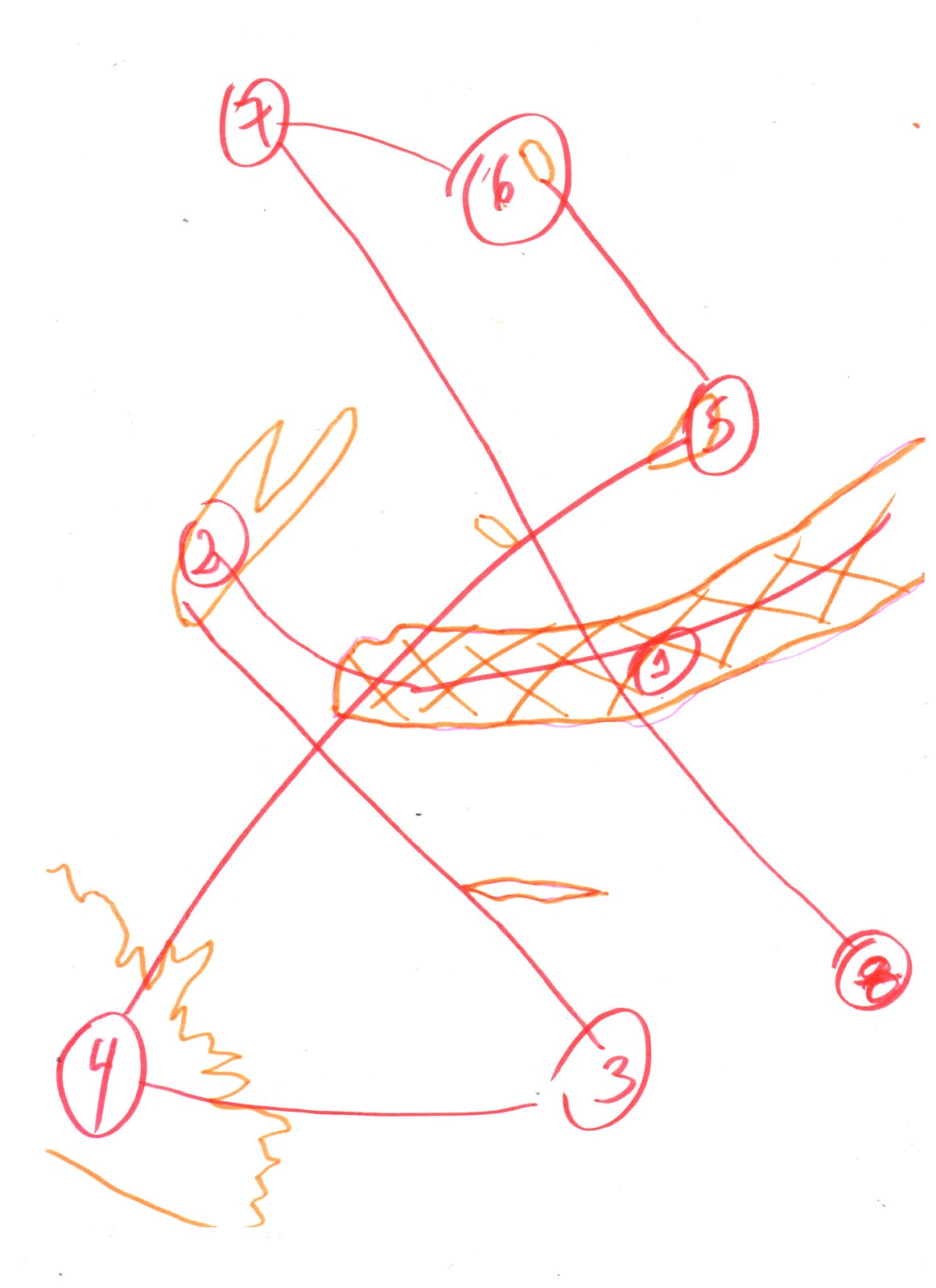This image is a complex drawing, possibly depicting a sequence of steps or a process. The diagram features numbered waypoints from 1 through 8, all connected by red lines that zigzag and cross over in multiple directions. Each number and line is illustrated in red, though there are also some orange elements present whose purpose is unclear.

The path begins at point 1, located near the center-right of the image, and progresses to point 2 at the center-left. Following the sequence, point 3 is positioned at the center bottom, point 4 is at the bottom left, point 5 is near the center, slightly to the right, point 6 is at the center top, point 7 is at the top left, and finally, point 8 is found at the bottom right.

The intricate network of lines and numbers suggests a highly detailed process or instructional sequence, but its exact purpose remains ambiguous. The additional orange markings add another layer of complexity, leaving their significance open to interpretation.